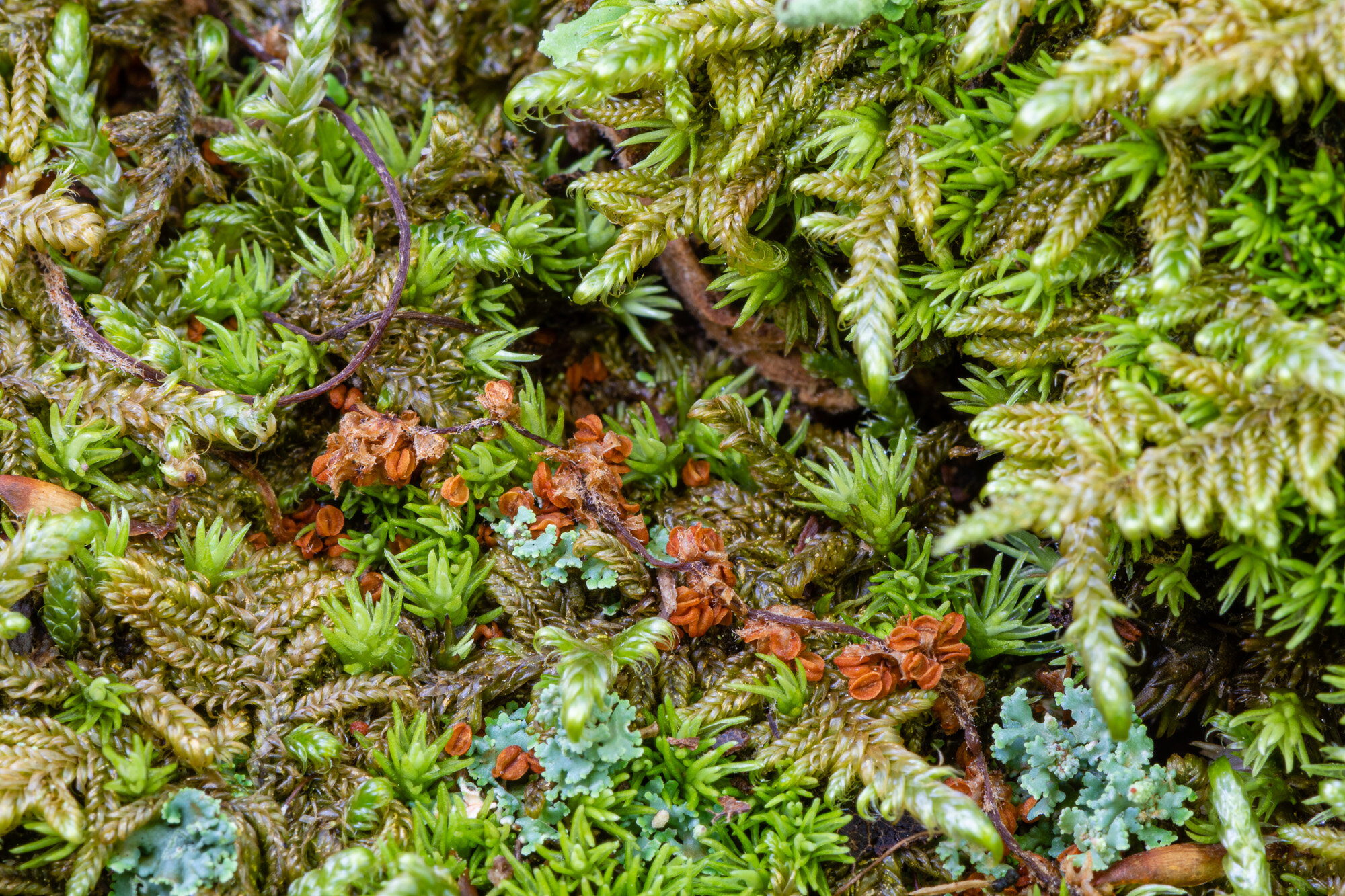This detailed close-up, color photograph captures a wild, intricate array of small, textured elements resembling leaves, stems, and bits of natural debris, set against an outdoor backdrop, likely taken during the day. The entire frame is filled with an eclectic mix of greenery and colorful accents, showcasing an assortment of plant-like fragments in various hues of green—ranging from light green to dark green and olive—interspersed with shades of brown, rust, and aqua. Among these are tiny vine-like strands, some of which are purple, and hints of orange, suggesting the presence of moss or algae. There are also pieces that appear blue. The ensemble comprises different types of plant leaves, twigs, berries, or possibly husks, all tangled together in a dense, mesmerizing mass. The photograph's close proximity to the subject matter creates a detailed and somewhat ambiguous view, highlighting the tiny, intricate structures and textures, which could be mistaken for woven fabric or yarn meant to resemble nature.